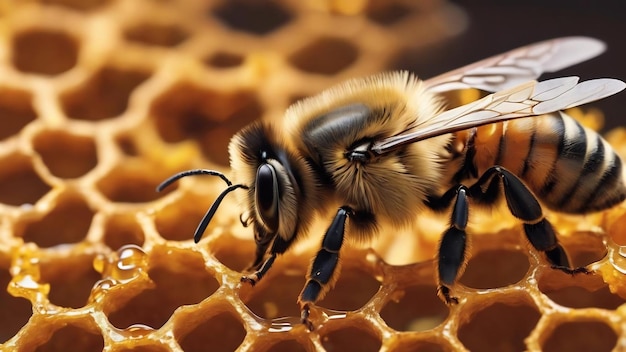A hyper-detailed, digitally stylized macro image showcases a honeybee from a close-up perspective, enhancing its intricate details to an almost surreal degree. The bee is perched on a honeycomb, characterized by its hexagonal patterns and dripping honey. Facing left and shown in profile, the honeybee's head is adorned with a furry, bright yellow ruff, framing two black antennae and a prominent single eye. Below its head, mandible-like structures reach into the honey. Its segmented body, marked by distinctive black and yellow stripes, leads to a black-colored tail. Six legs are visible, firmly grasping the honeycomb. The finely textured wings, translucent and light gray in color, lie flat against its back, originating just above the shoulder region. The foreground captures the bee and the honeycomb in sharp focus, while the background honeycomb fades into a diffuse blur, emphasizing the bee's vivid and detailed form.